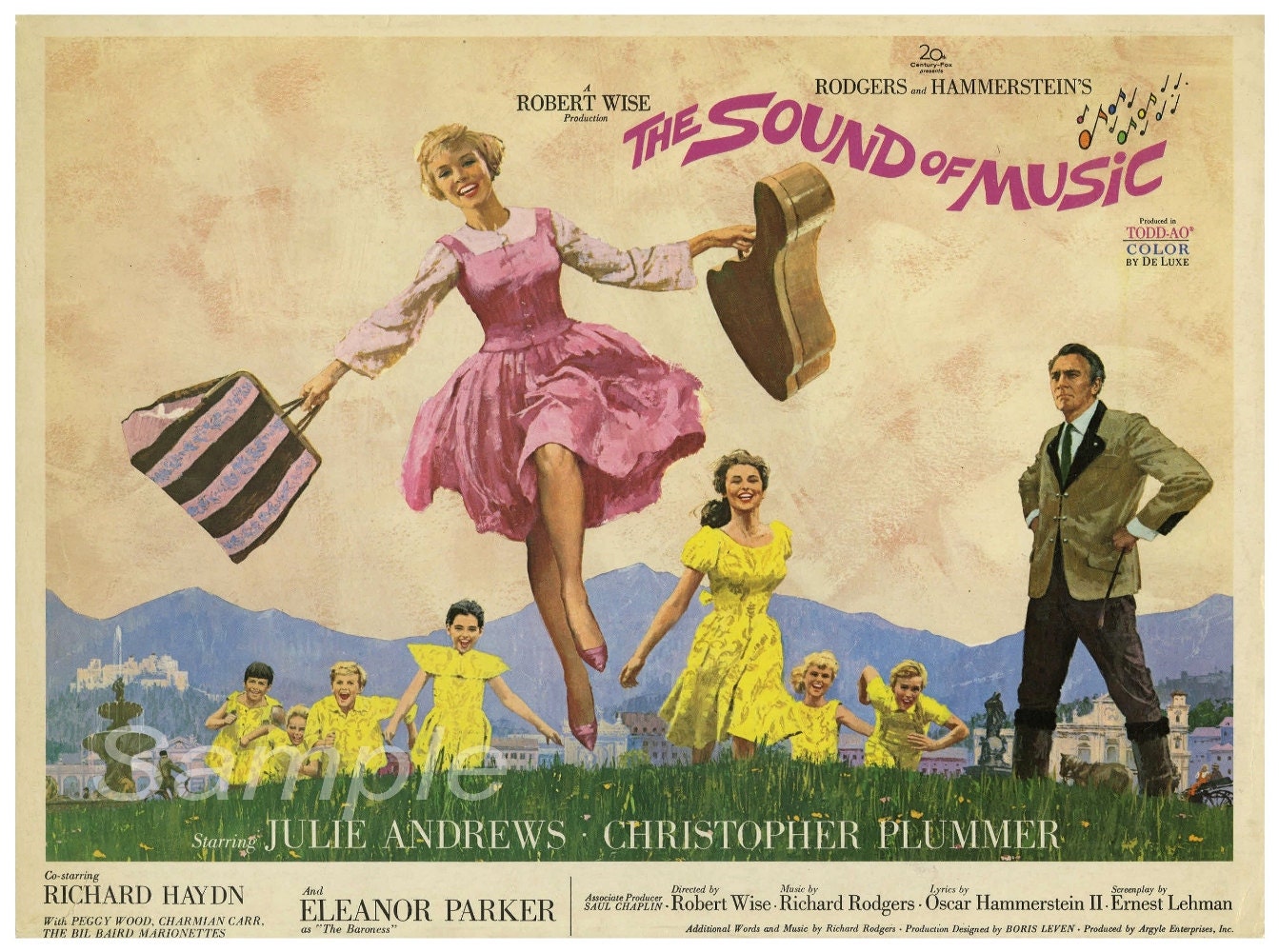This vintage movie poster for "The Sound of Music" prominently features Julie Andrews in the center, vibrantly depicted in a pink dress. She carries a guitar case and a striped black traveling bag while skipping joyfully through a picturesque meadow. Following behind her, the Von Trapp children, dressed in coordinating yellow outfits, dash through the grass. In the distance, Captain Von Trapp, portrayed by Christopher Plummer, stands with his hands on his hips, clad in a tie and suit coat, watching the scene unfold. The idyllic background showcases majestic mountains and a quaint village, enhancing the nostalgic charm of the image. At the top of the poster, musical notes dance around the bold title, "The Sound of Music," underlining it as a Robert Wise production proudly presented by 20th Century Fox. The names of the stars, Julie Andrews and Christopher Plummer, are prominently displayed, with additional credits at the bottom highlighting the significant contributions of co-stars Richard Hayden and Eleanor Parker. The poster's rich colors are noted as being rendered "by Deluxe," further emphasizing its timeless appeal and classic cinematic allure.